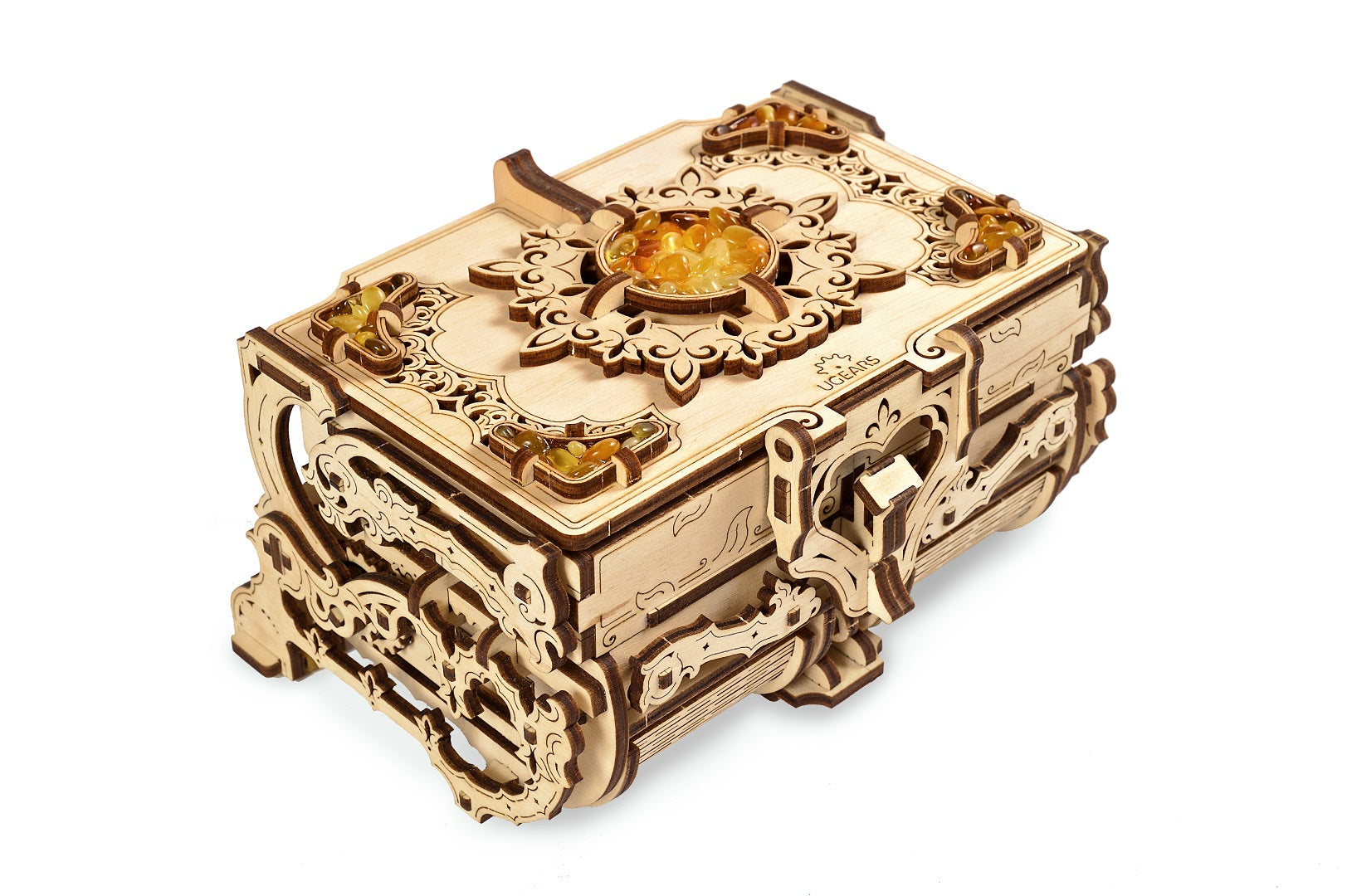The image showcases a highly ornate rectangular box, possibly a jewelry or treasure box, with intricate detailing. The box is predominantly ivory with brown accents and features extensive filigree woodwork on the sides. The surface appears golden and shiny, embellished with a floral pattern. The top of the box displays a circular arrangement of rough, translucent orange gemstones in the center, complemented by additional gemstones set in each corner within the wood filigree. The box boasts exquisite craftsmanship, with possible metal components and stenciled designs that contribute to its luxurious appearance. Notably, the lid is adorned with letters spelling out "U-C-E-A-R-S" against its elaborate backdrop.